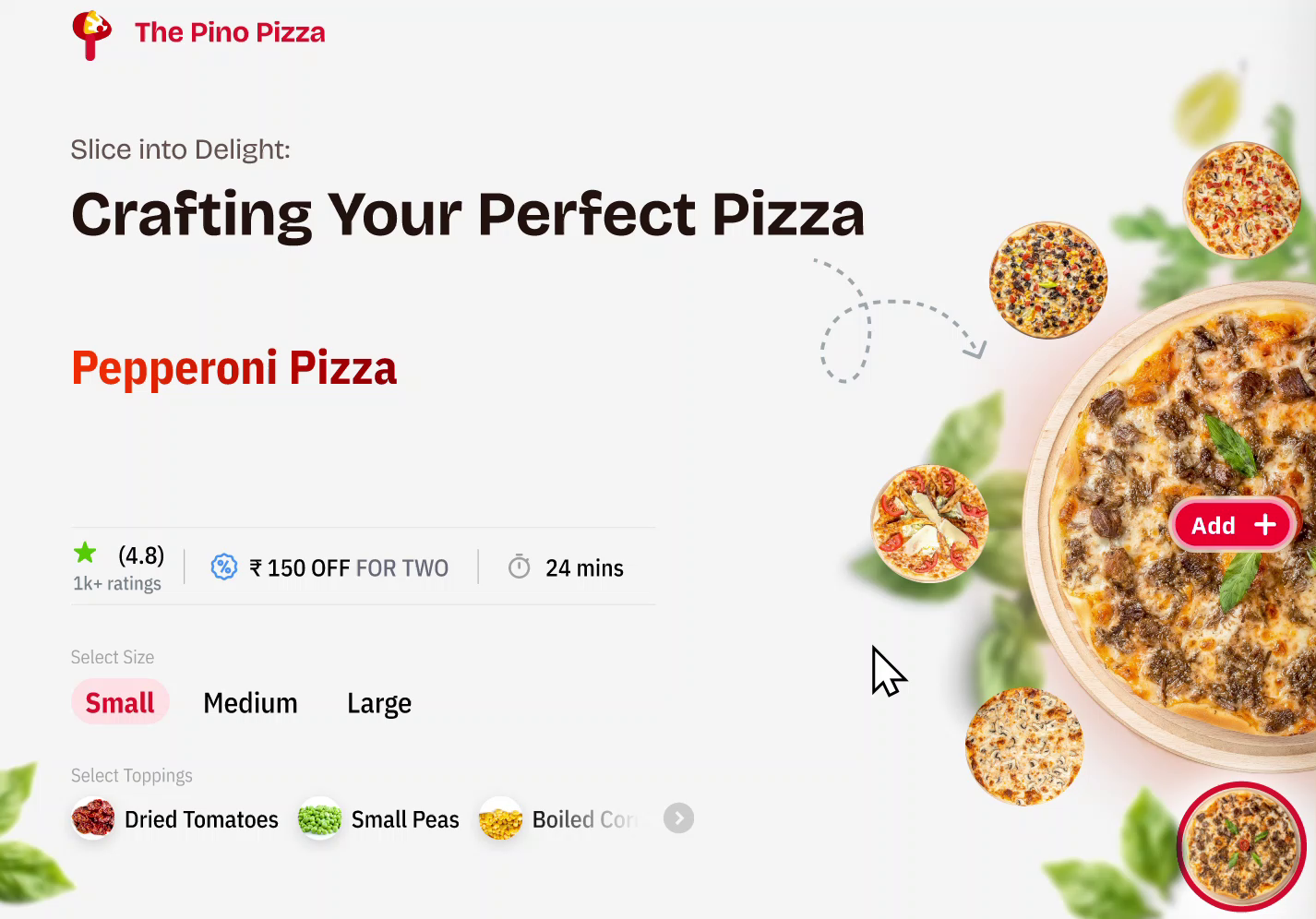Here's a cleaned-up and detailed caption for the image described:

---
**Pino Pizza Advertisement Screenshot**

The provided screenshot appears to be a web page advertisement for "Pino Pizza." In the upper left-hand corner, the text "Pino Pizza" is prominently displayed in red. Beneath this, the tagline reads "Slice into Delight" followed by "Crafting Your Perfect Pizza." The advertisement showcases a "Pepperoni Pizza" rated at 4.8 stars based on over a thousand ratings, likely out of five. A special offer is highlighted, stating "$1.50 off for two," with an estimated delivery time of 24 minutes.

The image allows users to choose from three pizza sizes: small, medium, and large. Additionally, three topping options are presented with circular photos: dried tomatoes, small peas, and boiled corn. On the right-hand side of the webpage, there's a larger picture of a pizza, surrounded by smaller circular images featuring different varieties of pizza with various toppings. 

Considering the detail and format, it might be from a different country, but this isn't clearly specified.

---

This caption provides a detailed and cleaned-up description of the features observed in the image.